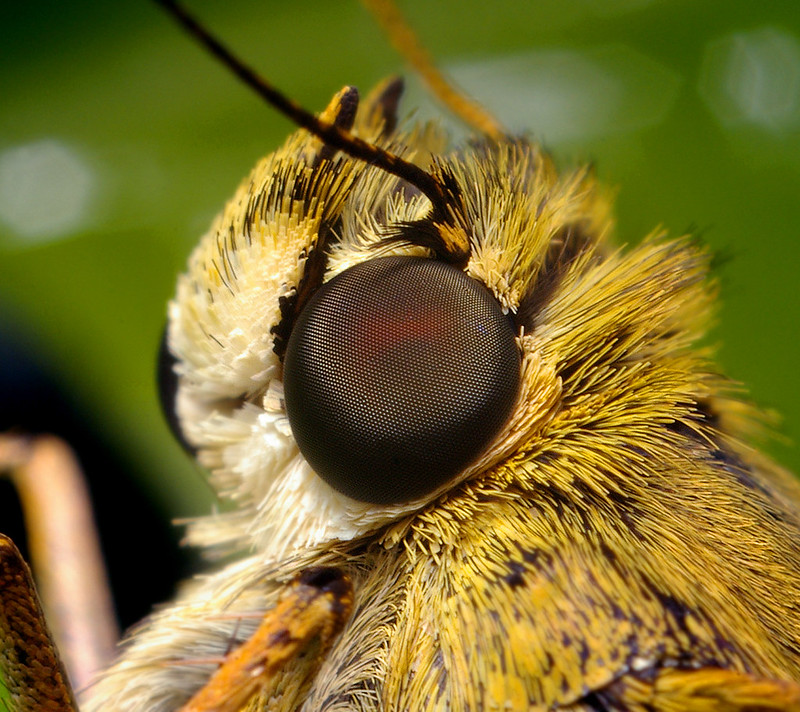This exceptionally detailed and vibrant close-up image captures a bee in stunning clarity, revealing details invisible to the naked eye. The photograph, taken outdoors against a blurred background of various shades of green, showcases the bee's head in profile as it appears to be perched on a leaf. The bee's eye is a prominent feature, large, round, and black, resembling a glossy button or small grape, with individual lines visible within the eye structure. The bee's body is covered in short, fuzzy fur-like hair, featuring a striking combination of yellow, white, and black. The face area between the eyes displays a lighter yellow hue. Two antennae extend from the bee's head, with the nearer one colored black and the further one yellow. Additionally, two of the bee's legs are subtly visible in the foreground of the image.